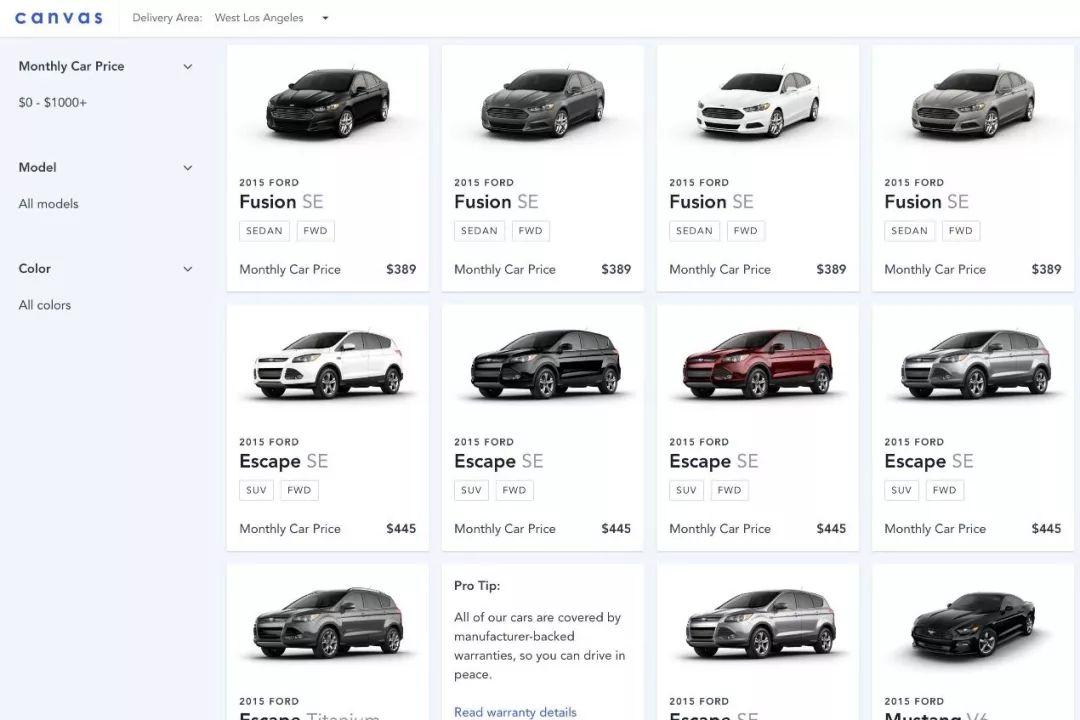This image represents a comprehensive car dealership website featuring a layout predominantly displaying various car models along with detailed information for potential buyers. The top-left corner prominently displays "Canvas" in blue, along with "Delivery Area: West Los Angeles." A blue vertical sidebar on the left provides filtering options including "Monthly Car Price: $0 to $1,000+," "Model: All Models," and "Color: All Colors," presented in black text.

The main section of the website is structured into a 4x3 grid, comprising a total of 12 boxes, 11 of which contain car images and their respective details. In the upper left box, there is a white rectangular area showcasing a black car with the following description: "2015 Ford Fusion SE Sedan, FWD (Forward Wheel Drive)," with a monthly car price of "$389."

In the second row, the leftmost box features a white SUV, labeled as a "2015 Ford Escape SE SUV, Four-Wheel Drive," priced at "$445" per month.

On the bottom left, another Ford vehicle is partially visible, though the specific details about this car are cut off.

Overall, this image indicates a user-friendly interface where customers can browse and filter car options based on their preferences such as price, model, and color.